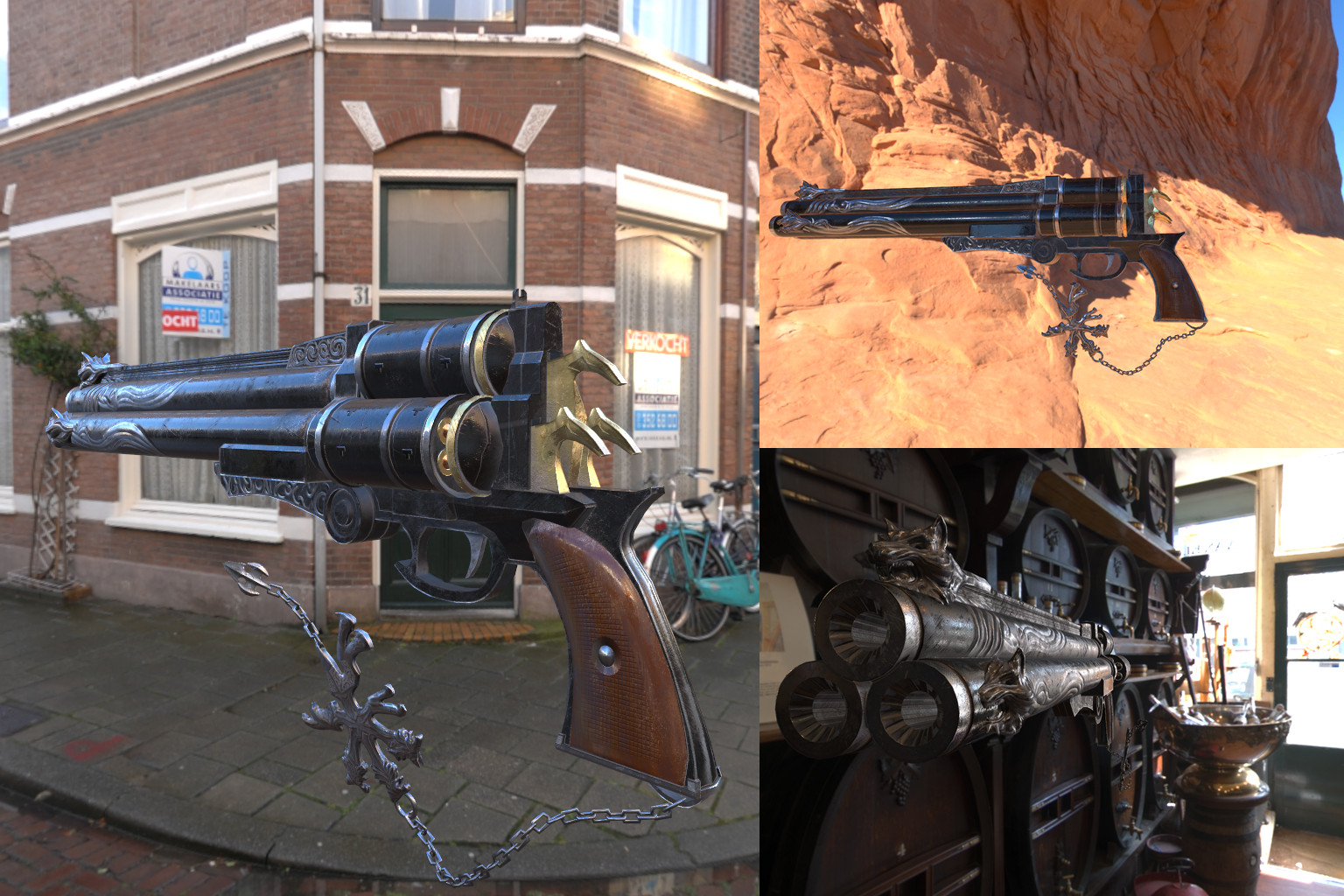The image style is graphic and is divided into three distinct sections. The left side, occupying two-thirds of the layout, features a steampunk-style revolver with three barrels and three triggers, floating as if photoshopped. This gun has a wooden grip and chains attached to both the grip and barrel tips. It's set against the background of a red brick corner building with white accents, including two white-framed windows and a door, which all sit under a visible arch and an additional story above. The sidewalk outside is grey and paved, and there is a blue bike leaning against the building. Two signs bearing the letters "OCHT" are visible on the windows.

In the top-right section, the same revolver is depicted against a striking brown and orange canyon backdrop with a slice of blue sky, highlighting the shiny black cylinders of the weapon.

The bottom-right section shows a three-quarter front view of the revolver, placed next to what appears to be a steam engine or some other piece of equipment. The grey barrels of the gun are prominently visible, and the setting includes a bowl and a window looking out onto the street, reinforcing the industrial, mechanical theme.